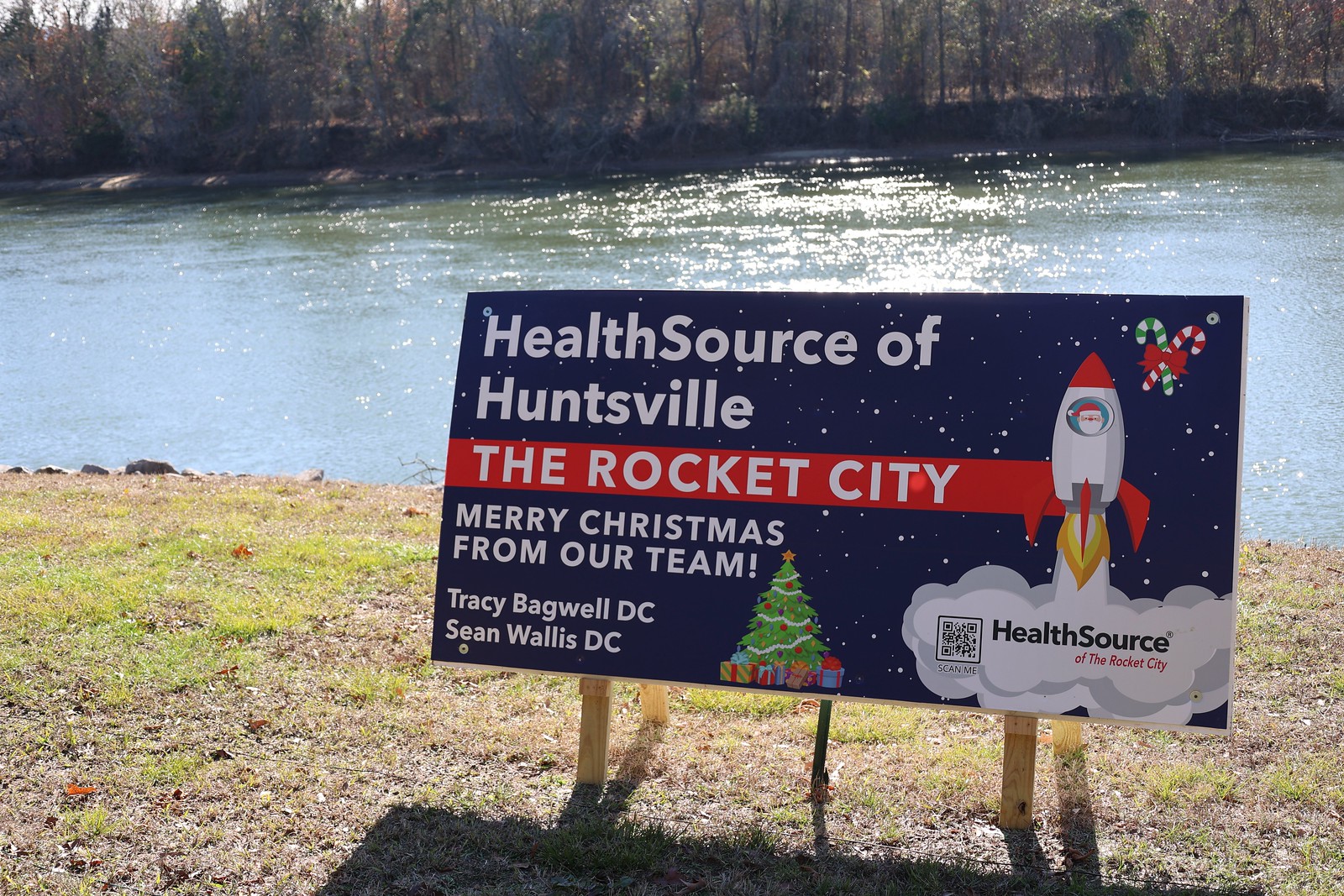This outdoor photo captures a festive sign positioned on a grassy mound in front of a small lake, with shimmering sunlight reflecting off the water. The lake is bordered by a densely wooded area on the far side, giving a serene, natural backdrop to the scene. The sign itself, rectangular and blue with white dots representing stars, is held up by wooden poles firmly planted into the ground.

The sign prominently reads, "Health Source of Huntsville, the Rocket City," in alternating text colors, with a secondary festive message below, "Merry Christmas from our team, Tracy Bagwell, D.C., and Sean Wallace, D.C." The bottom middle of the sign features a cheerful illustration of a Christmas tree surrounded by presents. In the upper right-hand corner there are candy canes tied together with a bow. Right below, Santa Claus is depicted peeking out of a rocket ship as it blasts off, leaving behind a trail of smoke that contains a QR code and the text "Health Source of The Rocket City." The picturesque setting and detailed holiday decorations create a charming and festive atmosphere.